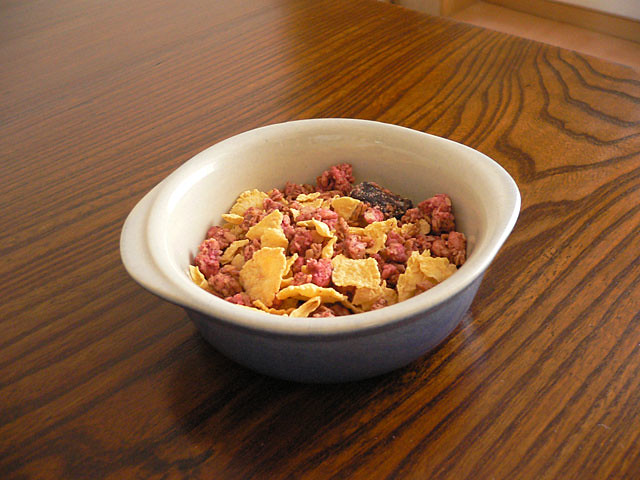A detailed caption for the image based on the shared and repeated details:

The photograph captures a white and light blue ceramic bowl, featuring two flanged lifting handles on opposite sides. The bowl, creamy white on the inside, contains a mix of breakfast cereals. The contents include light brown flakes resembling cornflakes, pink or reddish clustered pieces, and a few dark, possibly purple or chocolate-like items. The bowl is situated on a dark wood grain surface, which may be a tabletop or flooring, as the top right corner of the image reveals a baseboard or edge of a table next to a white wall. The ambiance suggests a kitchen setting, and despite the unusual cereal mix, it’s most likely intended for human consumption due to the presence of grains.